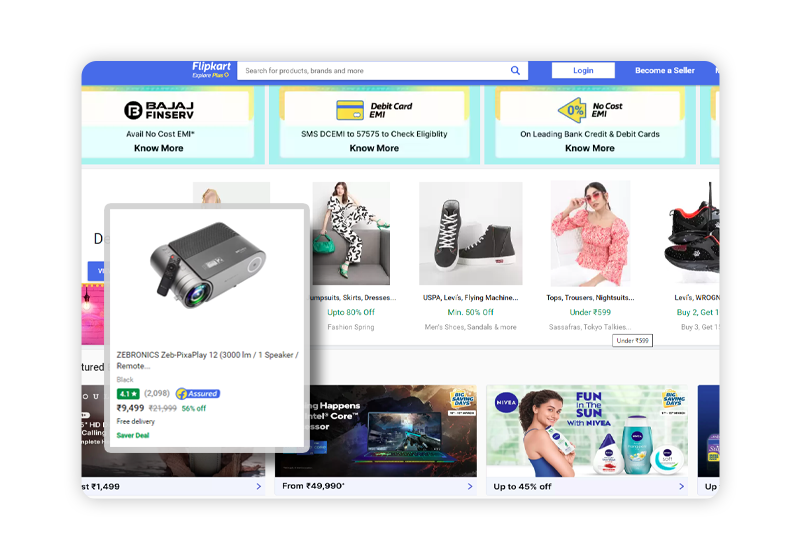A promotional image from Flipkart advertising a "No Cost EMI" offer in partnership with Bajaj and other brands. The image details several offers and products, such as a speaker with remote, free delivery, and discount deals starting from ₹4999. It also mentions various clothing items like tops, trousers, nightwalkers, and highlights brands like Levi's and Flying Machines. The EMI options are available on leading bank credit and debit cards with no additional cost.

In the visual, a woman is wearing a tank top and standing next to three distinctively shaped plastic bottles. 
1. The first bottle on the left is teardrop-shaped with a blue tip and a white body. 
2. The second bottle in the middle has a chunky, oval shape with a blue body and a white top. 
3. The third bottle on the right is round and white with a blue dot on the top and center, featuring a smiley face in a lighter blue color.

Another woman is dressed in a multi-colored floral outfit, resembling bell-bottom pants but as a shirt, with pink flowers on it, adding a vibrant and lively touch to the scene. The image encourages users to log in and search for more products and deals, with the tagline "Fun in the Sun with Nivea."